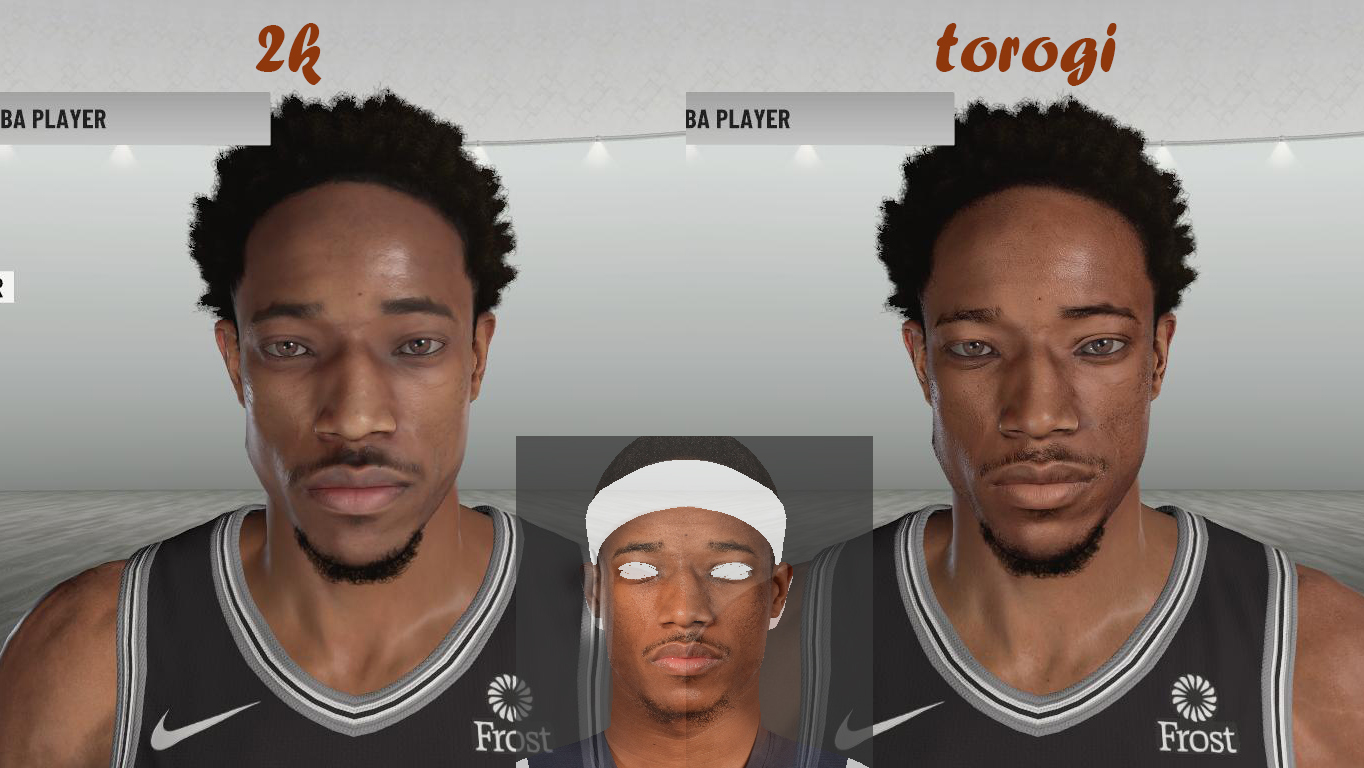A screen capture of a video game character customization screen, prominently featuring a horizontally-oriented gray banner at the top. On the left side of the image, just above a man's head, the red "2K" logo stands out. This man, likely in his late 20s, is depicted wearing a black jersey with a white Nike logo on the upper right shoulder and a circular white emblem on the left shoulder that reads "Frost" underneath. An identical character stands on the right with some variations in facial features. Above this character, the name "Tarogi" is displayed in a brownish-red hue. Both characters have matching hair, eyebrows, eyes, nose, mustache, and beard. Between them, a gray box showcases a base character face with a missing-eyed, white headband-wearing visage that is nearly identical to the other two characters except for the different hair and unsettling solid white eyes.